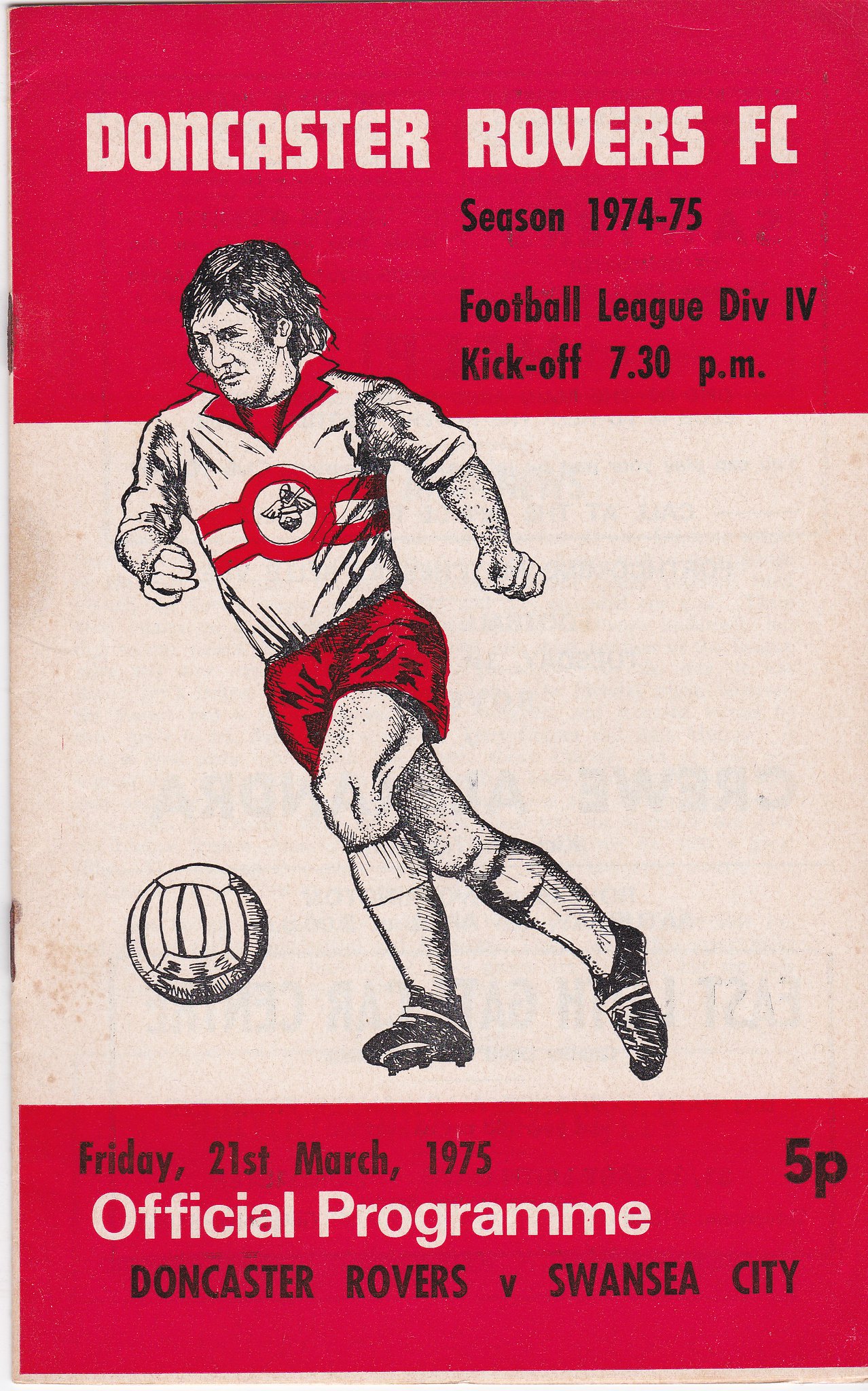This is an old soccer program poster from a match between Doncaster Rovers and Swansea City, dated Friday, March 21, 1975. The poster features a detailed pen-and-ink drawing of a soccer player dribbling, with dark hair and red shorts, a white shirt with a red collar, and black shoes. The player is positioned against a background divided into three sections: the top third and bottom third are red, while the middle portion is white. The team's emblem is displayed prominently on the player's chest.

At the top of the red section, "Doncaster Rovers FC" is written in white print, followed by "Season 1974-75" in black print. Below this, it states "Football League Division 4" and "Kickoff 7:30 PM" also in black print. Additional text includes "Official Programme" in white print, "Friday, 21st March 1975" and "Five Pence" in black print, and "Doncaster Rovers vs Swansea City" at the bottom. The ball is depicted slightly above the player's left foot, adding to the dynamic nature of the illustration.